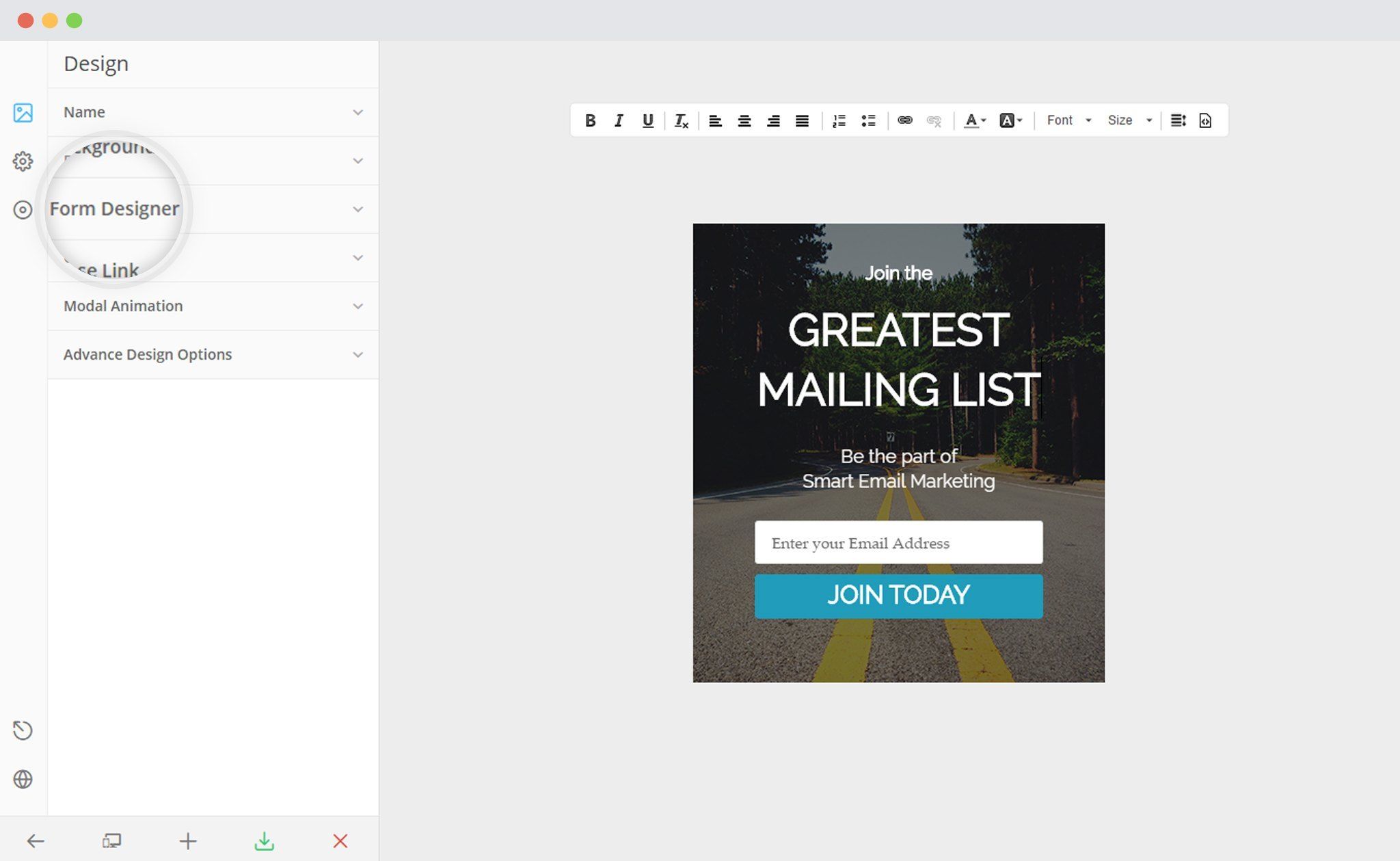This image appears to depict an application on an Apple device. In the top left corner, there are three circular buttons: a red circle, a yellow circle, and a green circle, typical of window controls on macOS. Below these controls, a sidebar menu lists several categories in a vertical sequence: "Design," "Name," "Background," "Game Designer," "Link," "Model Animation," and "Advanced Design Options." Each of these categories has a downward-facing arrow to its right, suggesting expandable menus or filters.

On the far left side, the sidebar also features various icons: a picture icon colored in blue at the very top, followed by a gear icon beneath it, and a double-circle icon below the gear. Further down, there is a globe icon at the bottom left corner, and just above it sits a power button icon.

Dominating the middle-right section of the image is a photograph with text superimposed on it. The text reads, "Join the Greatest Mailing List, Be Part of Small Email Marketing," in white font. The background of this photograph features a road with two yellow stripes running down the middle, flanked by lush green forest on either side.